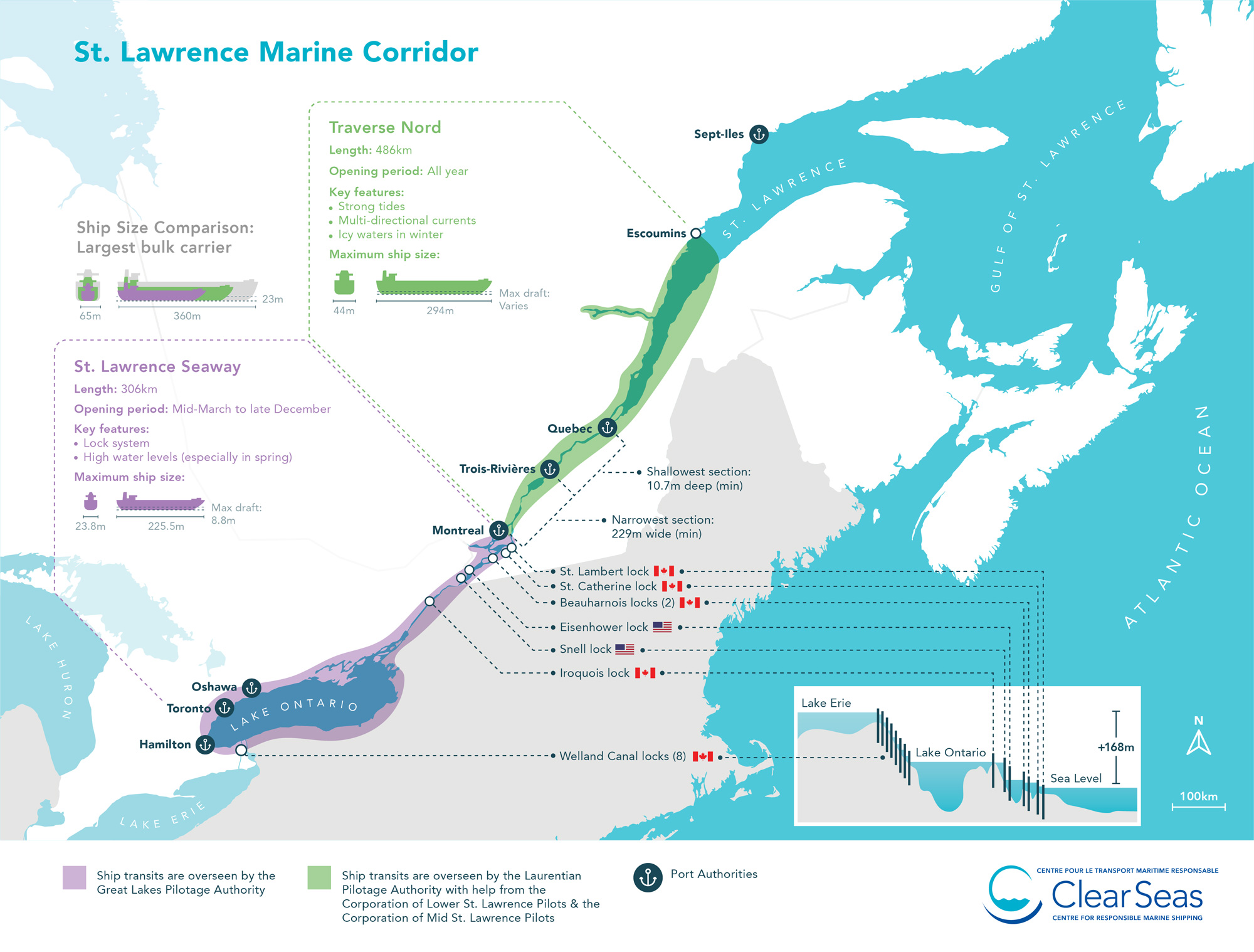This is a highly detailed and visually rich map of the St. Lawrence Marine Corridor, created by Clear Seas. The map covers various bodies of water, including the Atlantic Ocean, Gulf of Lawrence, St. Lawrence River, Lake Ontario, and Lake Erie. It features a multitude of colors—blues, purples, greens, and whites—to depict different regions and their overseeing authorities such as the Great Lakes Pilotage Authority and the Laurentian Pilotage Authority. Highlighted within the map are sections dedicated to the Green Traverse Nord and the St. Lawrence Seaway, including detailed information about ship size comparisons, such as large bulk carriers, and the St. Lawrence Seaway's length, opening period, and key features. The map also displays critical maritime infrastructure close to Lake Ontario, such as the St. Lambert Lock, the St. Catherine Lock, the Behemoth Lock, the Eisenhower Lock, the Small Lock, the Iroquois Lock, and the Whalen Canal Locks. Surrounding areas are indicated with cities like Oshawa, Toronto, and Hamilton. Additional text provides insights into sea levels, the Marine Corridor's key features, and specific views, both front and side, of large ships navigating through areas like Traverse Nord.